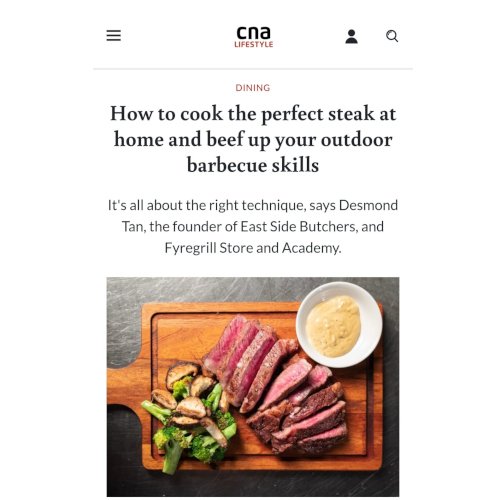This image captures a mobile view of an article on CNA Lifestyle, featuring the section titled "DINING" in bold, red, all-capital letters, just below a faint green line. The main headline, "How to Cook the Perfect Steak at Home and Beef Up Your Outdoor Barbecue Skills," is prominently written in a larger black font. The article quotes Desmond Tan, the founder of Eastside Butchers and Fry Grill Store and Academy, emphasizing that achieving the perfect steak is all about the right technique.

At the bottom of the image, a rustic wooden cutting board with a long handle and an indented edge to hold juices is displayed. Positioned on the cutting board is a creamy, yellowish-tan sauce in a small bowl resting in the upper right corner. The board also features several pieces of high-quality beef, possibly filet mignon, artfully arranged in clumps. Accompanying the beef are assorted vegetables and mushrooms, adding a burst of color and texture to the enticing scene.